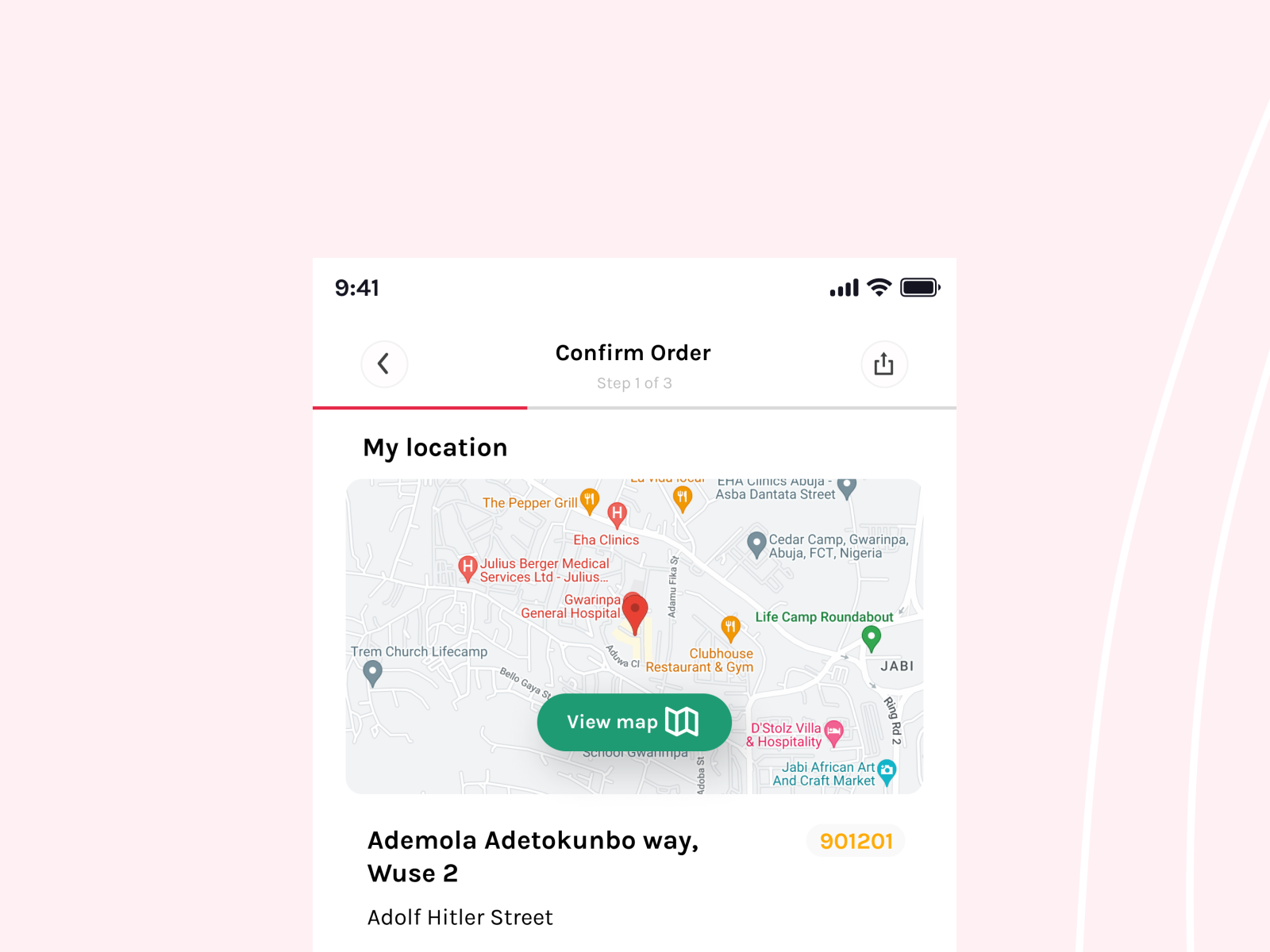This screenshot, captured on an iPhone, showcases a delivery or map application. The phone's interface indicates the time is 9:41 AM, with the top right corner showing a nearly full battery and a Wi-Fi connection. The background of the app is light gray with two horizontal lines on the right side. The app is in 'Confirm Order: Step 1 of 3', featured prominently at the top of the screen, albeit slightly faded. Below this, there's a share icon on the right and a back arrow on the left. The map displayed illustrates various rows and icons, marking locations such as restaurants, gyms, and other services. A green 'View Map' button and a 'my location' icon are also visible. At the bottom of the screen, the street and zip code (901201) are shown, along with specific locations like Adomola Adotokubo-Wei and amusingly, Adolf Hitler Street.